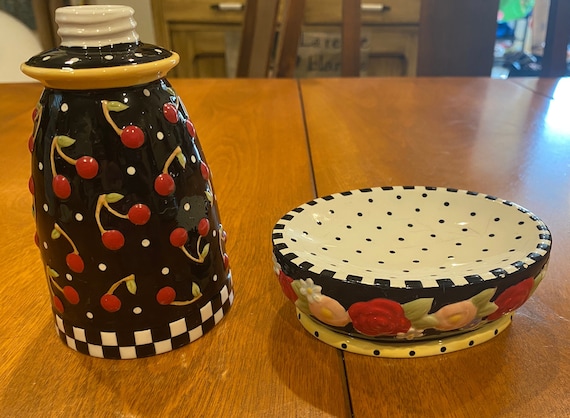The photograph captures two porcelain objects positioned on a light yellowish-brown wooden surface, likely in a kitchen setting. The object on the left is a tall, black jar adorned with a vibrant cherry pattern—red cherries with green stems and leaves—set against a black and white checkerboard base. This jar might have a screw top and resembles Mary Engelbrecht’s whimsical artwork. On the right side of the image sits a matching bowl. The bowl’s interior is white with black polka dots, with a black checkerboard rim, and it features colorful roses—red and yellow with green leaves—around the bottom. Both pieces showcase intricate, complementary designs and stand out against the indistinct background, which hints at a domestic space with visible cabinets and a door.